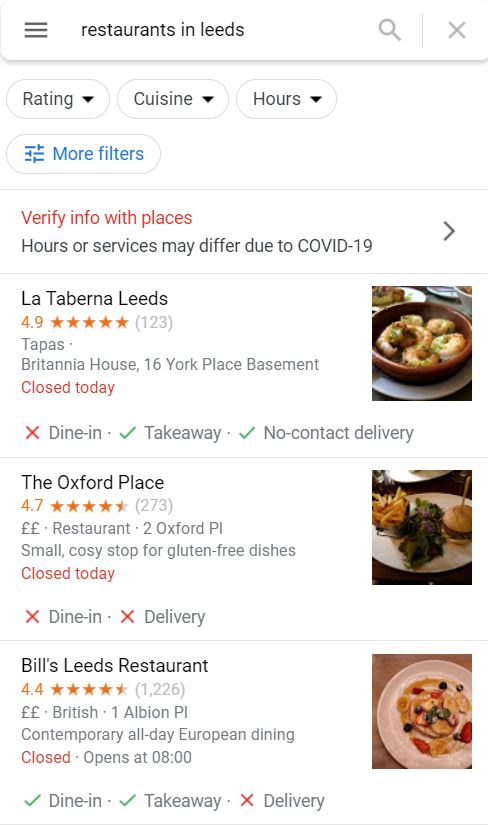Screenshot of a Google app search for restaurants in Leeds, United Kingdom, showing results with detailed information. Below the search bar are tabs for sorting by "Rating," "Cuisines," and "Hours," along with an additional "More filters" option. A red notification advises users to "verify info with places." 

The results list four restaurants:

1. **La Taberna Leeds**
   - **Rating:** 4.9 stars from 123 reviews
   - **Cuisine:** Tapas
   - **Address:** 16 York Place Basement
   - **Status:** Closed today (in red text)
   - **Services:** Takeout and no-contact delivery only; no dine-in
   - **Image Description:** A dish from La Taberna

2. **The Oxford Place**
   - **Rating:** 4.7 stars from 273 reviews
   - **Price Level:** ££
   - **Address:** 2 Oxford Place
   - **Status:** Closed today (in red text)
   - **Services:** No dine-in or delivery options
   - **Image Description:** A hamburger served with fries and some salad

3. **Bill’s Leeds Restaurant**
   - **Rating:** 4.4 stars from 1,226 reviews
   - **Price Level:** ££
   - **Address:** 1 Albion Place
   - **Status:** Opens at 8 AM (in red text)
   - **Services:** Offers dine-in and takeaway; no delivery
   - **Image Description:** Pancakes topped with sliced strawberries, bananas, blueberries, and syrup